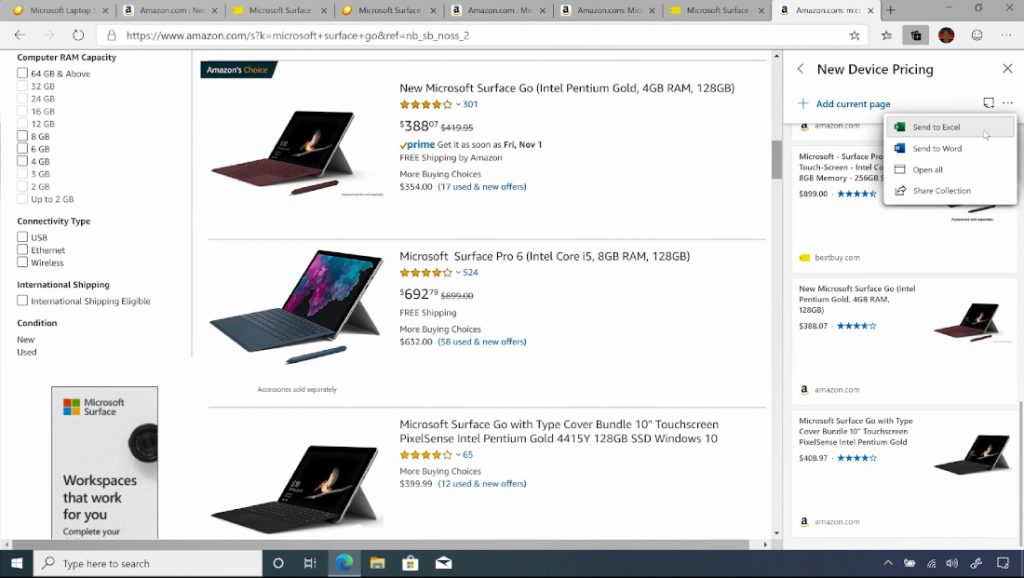The image displays a screenshot of a desktop screen with a web browser open to the Amazon website. At the top of the browser, a grey band indicates that there are eight tabs open. Directly below this, the URL bar confirms the site being viewed is Amazon. The user is conducting a search for computers or laptops.

On the left side of the page, there is a filter menu allowing users to refine their search based on various criteria such as capacity and connectivity. In the central area of the page, several computer listings are visible. Each listing includes a product image, the name of the computer, its rating, a brief description, and the price. The screenshot specifically shows three such computer listings.